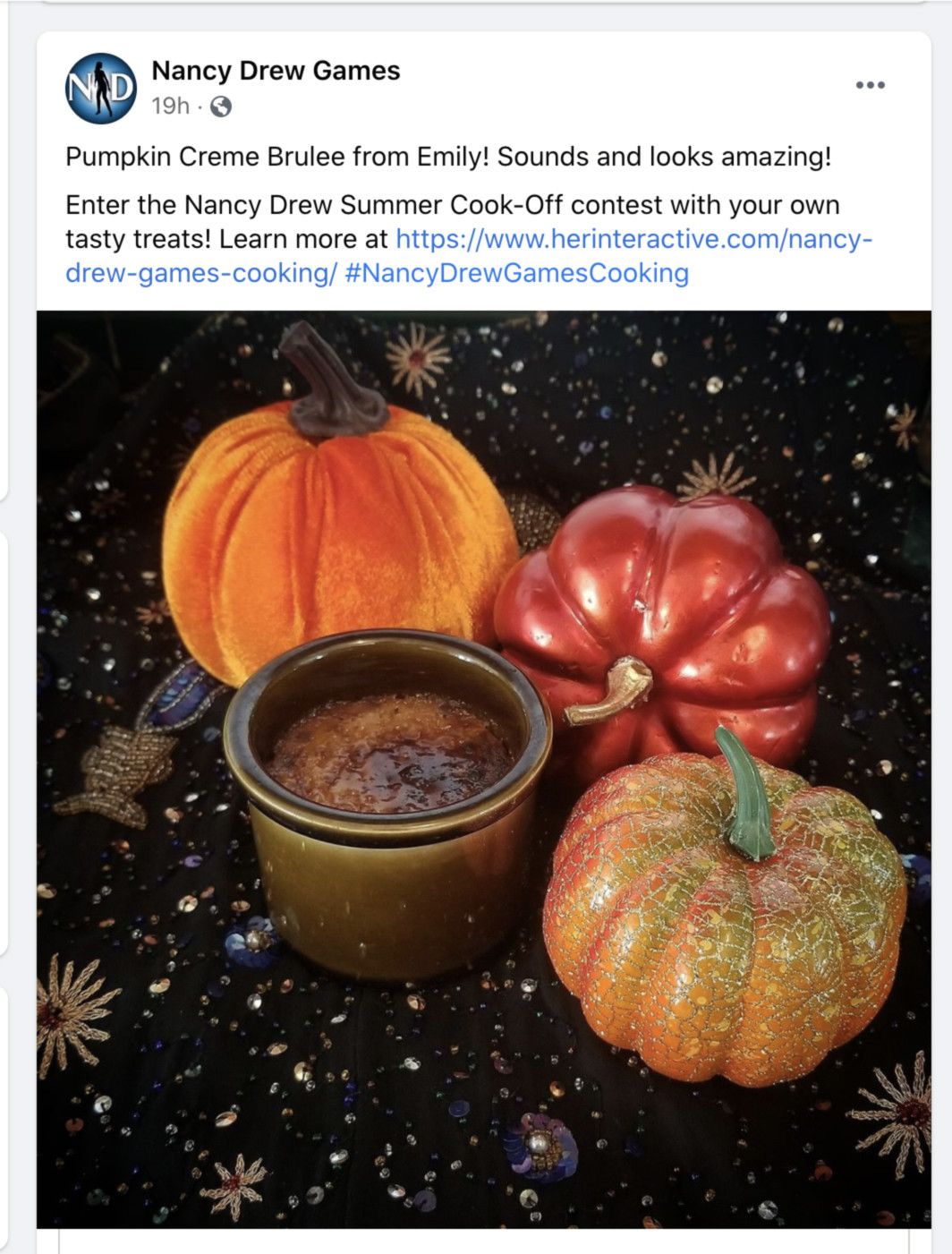The web page prominently features a game-themed layout with blue banners framing the sides and top. The central banner, stretching horizontally, displays an insignia on the left side: an oval with a blue background, a white "N" on the left, and a white "D" on the right, enclosing a black silhouette of what seems to be a woman. Adjacent to this insignia, in bold black letters, are the words "Nancy Drew Games."

Beneath this, in a lighter gray color, it reads "19H" followed by a dot and what appears to be a small globe symbol. Further down, in dark gray or black text, there's an enthusiastic message: "Pumpkin cream brûlée from Emily! Sounds and looks amazing!" accompanied by a call to action: "Enter the Nancy Drew Summer Cook-off Contest with your own tasty treats." An invitation to "Learn more at" followed by a bright blue web address completes the textual information.

Below the text is an illustration or painting rather than a photograph. This artistic representation features a dark gray tablecloth adorned with various flowers. On the top left-middle of the image is an orange pumpkin, while the top right-middle showcases an orange-bronze squash. In front of these elements, there’s a cut-off pumpkin lid with an attached stem, displaying hues of light orange and green. Central to the illustration sits a brown, metallic-looking plate containing what is presumably the pumpkin cream brûlée mentioned in the introductory text.